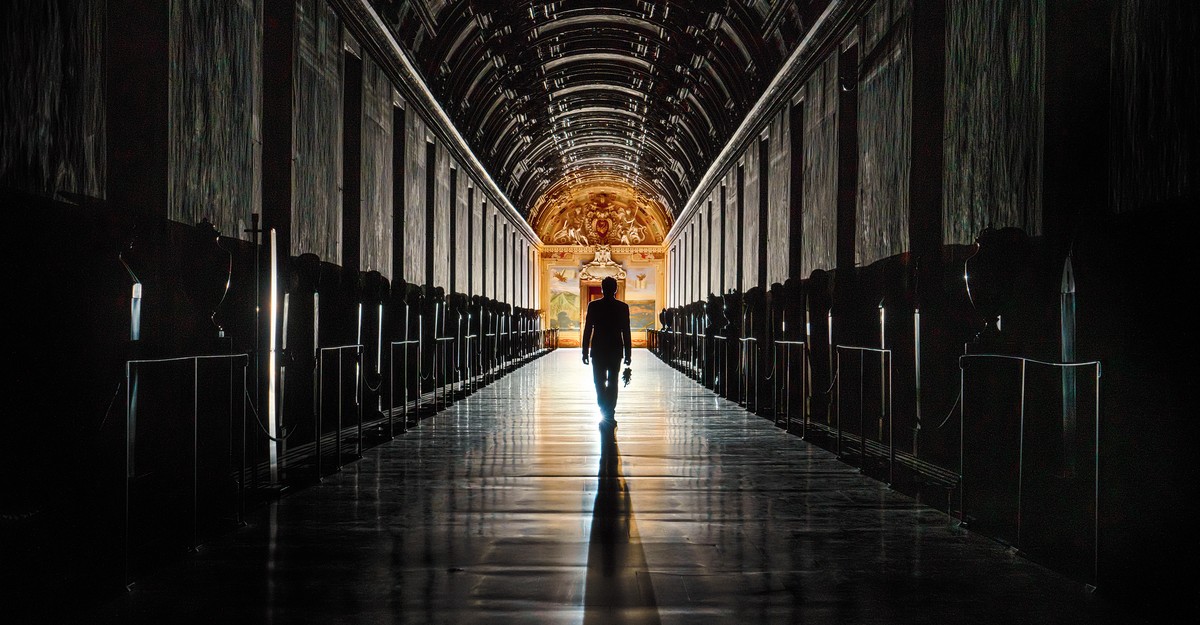In this photograph, a man is walking forward through a dimly lit church, his back to the viewer, casting a shadow on the dark walls around him. The church's interior is predominantly cloaked in darkness, with nearly black walls and a round, black ceiling adding to the somber atmosphere. This stark contrast is broken by a vibrant orange wall at the end of the hallway, adorned with intricate gold features that reflect onto the polished floor, providing the only source of light and color in the scene. The man, who appears to have short hair and is of average height, holds an indistinguishable object in his right hand as he walks towards what seems to be an altar or a significant point of focus, illuminated from behind. Adding to the rich detail, both sides of the hallway feature crosses and objects resembling urns, likely adding to the religious and ornate character of this church setting.